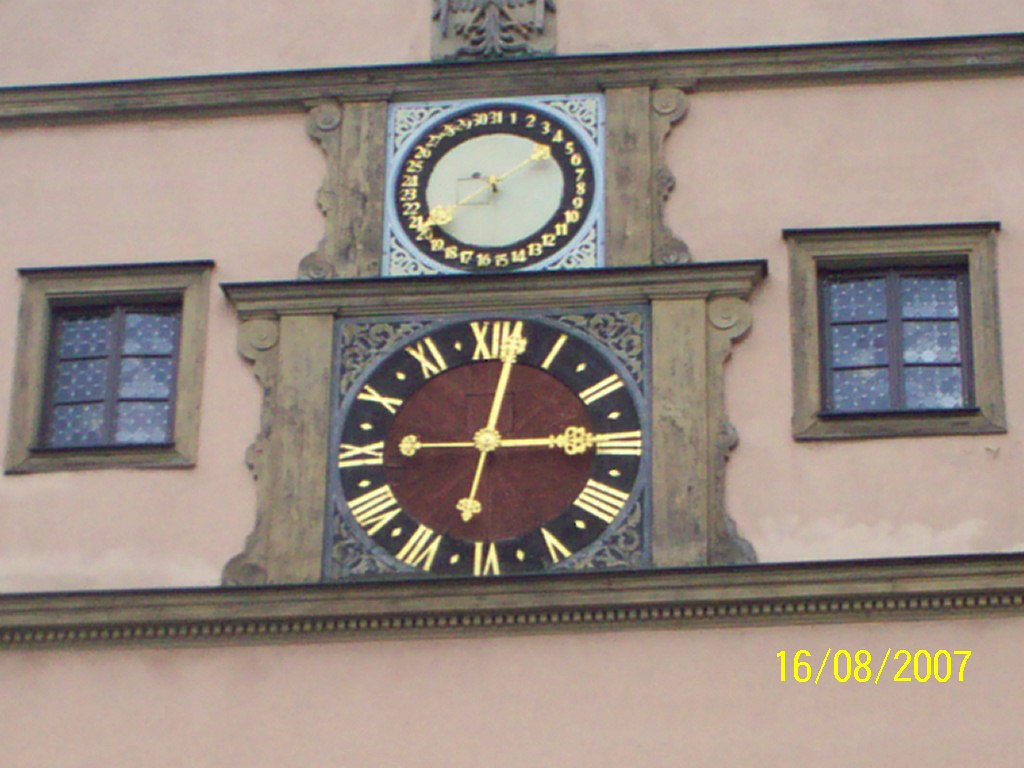The image depicts two stacked clocks mounted on the side of a beige, plastered building, nestled between two windows that are covered by blue blankets or curtains, obscuring any view into the interior. The top clock is smaller, featuring a black outer rim, a gray inner face, and a single golden hand, displaying a calendar with numbers ranging from 1 to 31. The larger, bottom clock has a black rim encircling a reddish face marked with Roman numerals. It possesses golden minute and hour hands, both distinctive against the vintage backdrop. The careful arrangement and detailed design of the clocks contrast with the simplicity of the building’s facade.